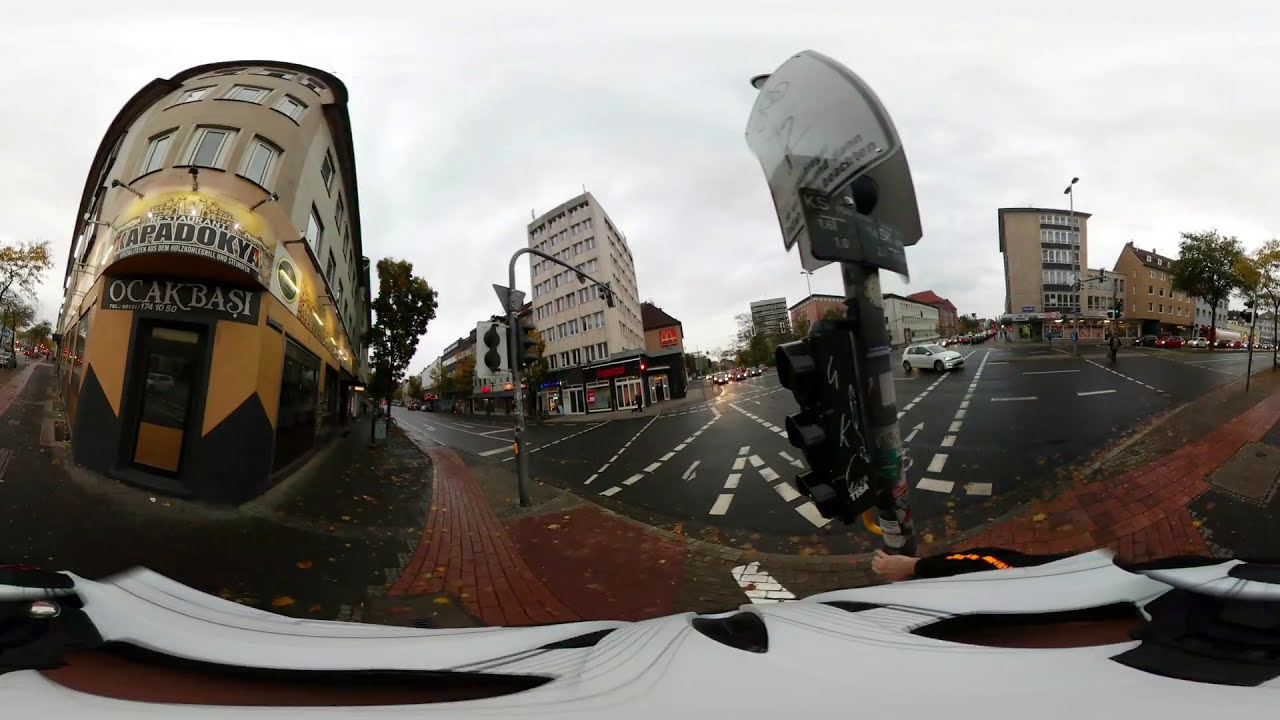The image is a 360-degree fisheye view of a city street, likely in a Middle Eastern or European city, creating a skewed effect where some objects appear larger or smaller than usual. Starting on the left side, there is a three-story white building with a storefront featuring a prominent yellow and black entrance. Above the door, the storefront displays two signs: one reading "OCAKBASI" (Okakbasi) and another above it spelling out "KAPADOKYA". The word "restaurant" is also visible. The storefront is adorned with lights that are turned on despite the overcast daylight. Nearby, trees line the cobblestone sidewalk. 

The street in front features white dashed lines and multiple cars, including a white car emerging from behind a black traffic light. There are several additional buildings, including a five or six-story one that appears to be either offices or apartments. A McDonald's is centrally located, identifiable by its iconic arch sign. Pedestrians are scattered along the street, and a crosswalk is directly in front of the image. Traffic signals and street signs, although slightly skewed due to the fisheye lens, contribute to the bustling atmosphere of the urban street scene.